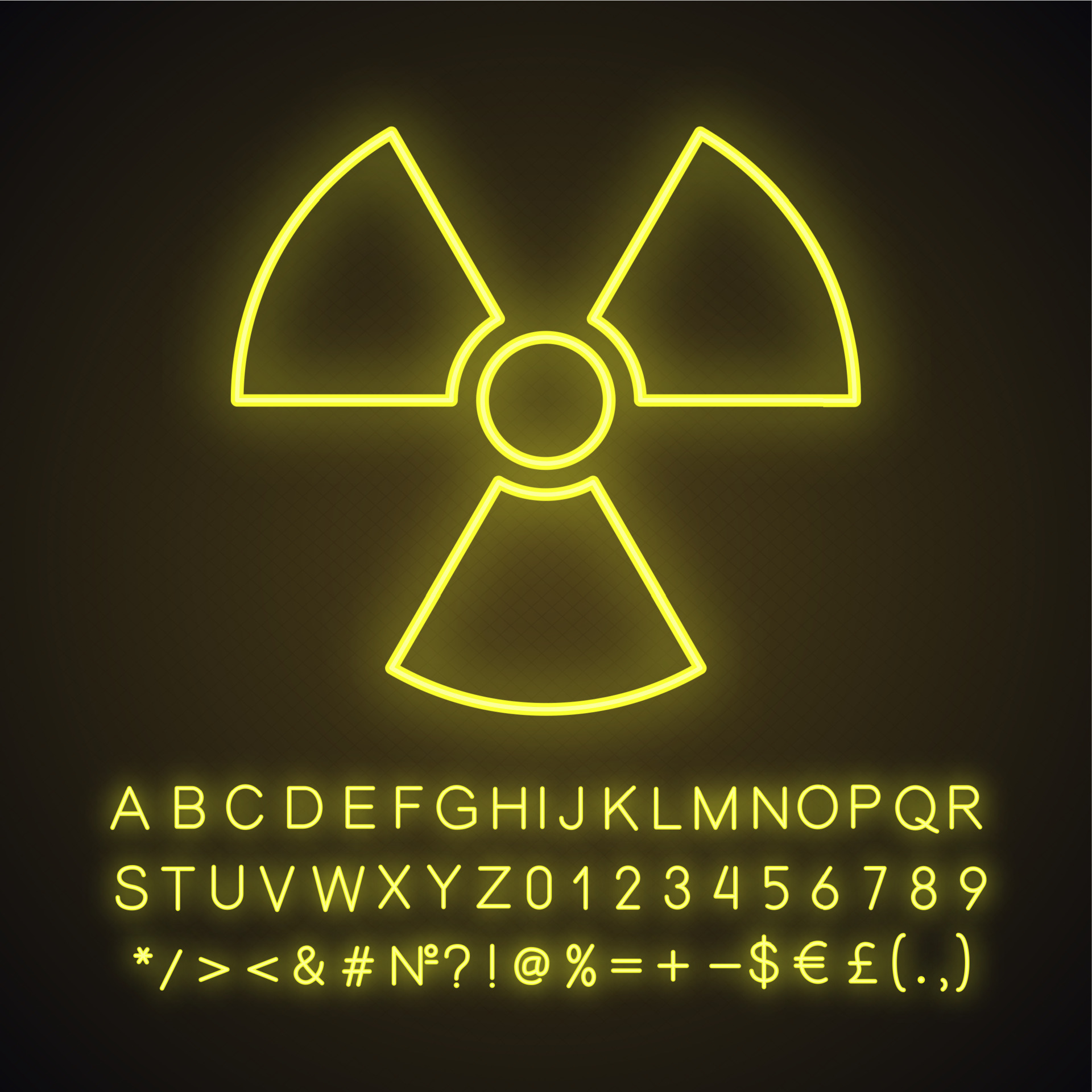The image showcases a neon yellow warning sign set against a completely black background. At its center is a glowing yellow circle, surrounded by three equally spaced, truncated triangular shapes, resembling the radiation hazard symbol. Below this emblem, the alphabet is displayed in capital letters in two lines: A through R on the first line and S through Z on the second. Directly beneath the alphabet, the numbers 0 through 9 are listed in the same vibrant yellow hue. At the bottom of the image, an array of keyboard symbols, including ampersands, arrows, slashes, dollar signs, and pound signs, can be found. The entire composition is highly luminous and visually striking, with no other colors present.